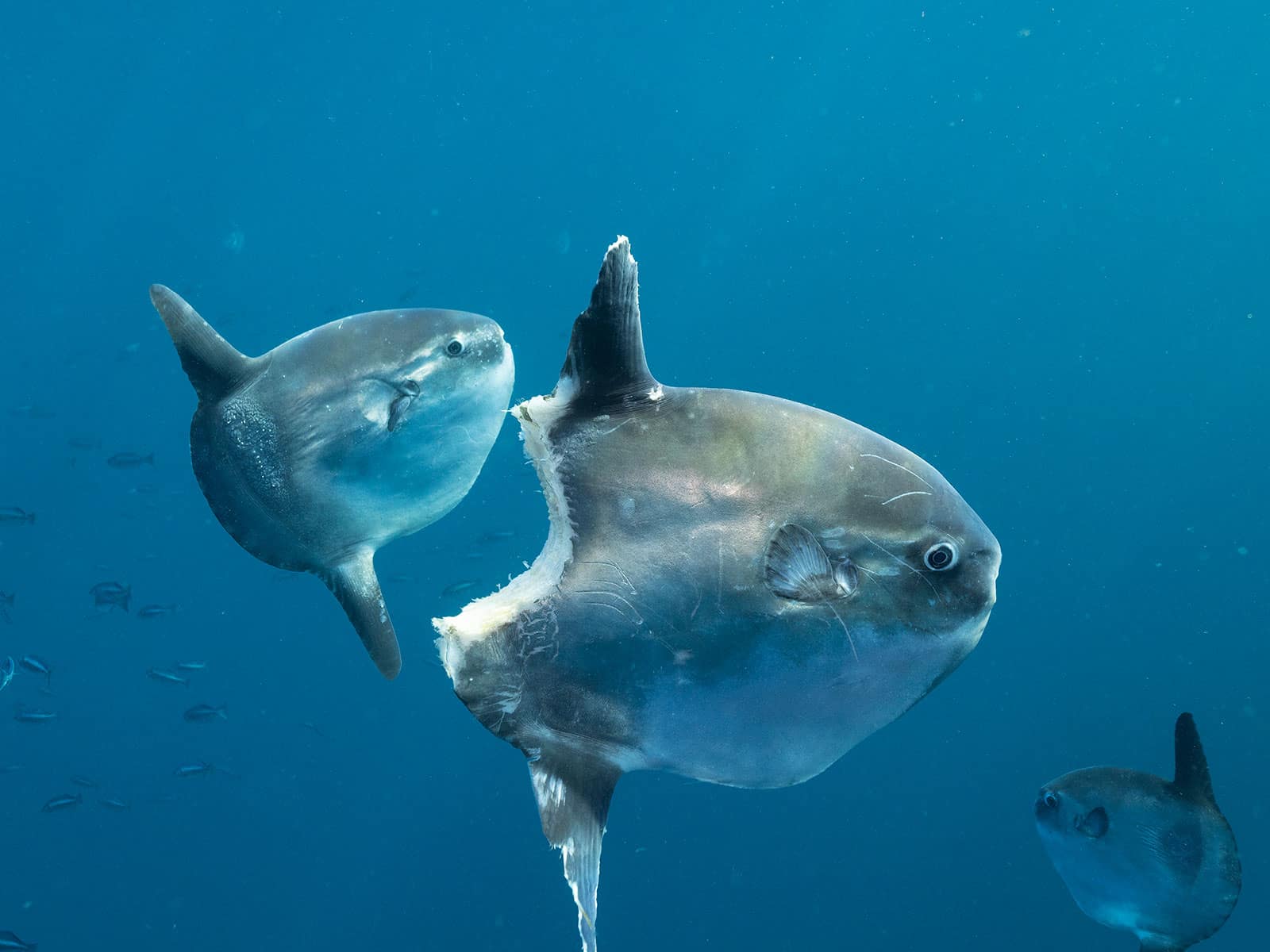In this striking underwater photograph, the dark blue water is speckled with white, setting the scene for the three prominent, oval-shaped fish that dominate the image. Positioned in the center, left, and bottom right of the frame, these dark gray fish exhibit a blend of characteristics reminiscent of pufferfish, sharks, and anglerfish. Each possesses top and bottom fins, along with a side fin and a visible eye on their flat sides. The central fish is the most arresting; it has endured a massive bite out of its backside, exposing stark white flesh and creating a jagged, curved wound. Despite this gruesome injury, the fish appears to still be alive. The other two fish remain intact, with one situated towards the bottom right and the other on the left, near smaller fish swimming in the background. This image’s surreal quality, coupled with the bizarrely grotesque injury of the central fish, raises questions about its authenticity, suggesting it might be AI-generated.